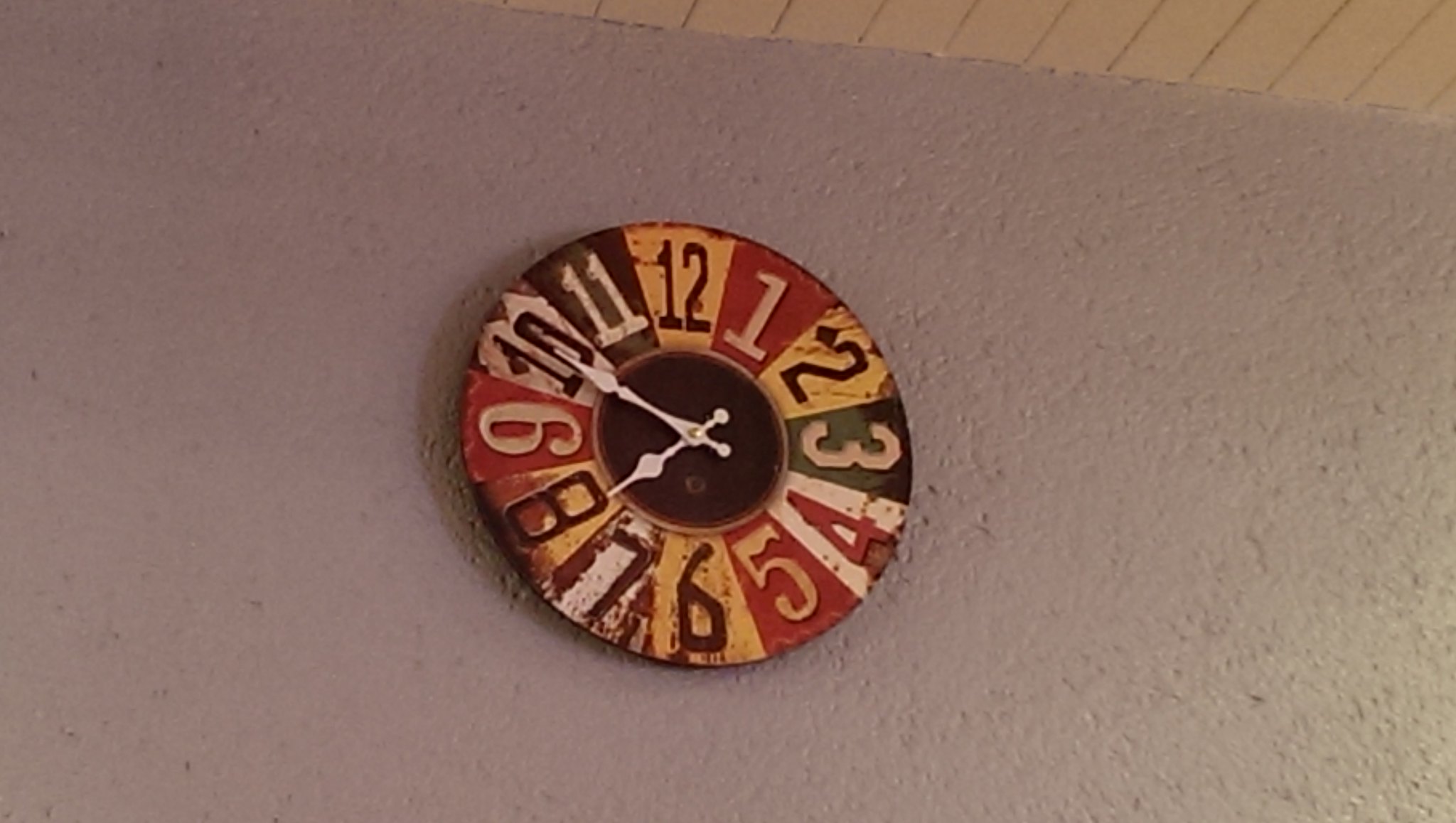A vividly detailed, multicolored clock is showcased in this image, lying on a textured concrete floor with visible paneling around it. The clock face features distinct sections of yellow, red, and green, with alternating black and white numerals based on their position. Adding to its charm, the clock has white hands that taper to fine points, indicating the time as ten minutes to eight. The inner circle of the clock is intentionally distressed, showcasing purposeful chips, faded areas, and worn spots, contributing to its vintage aesthetic.